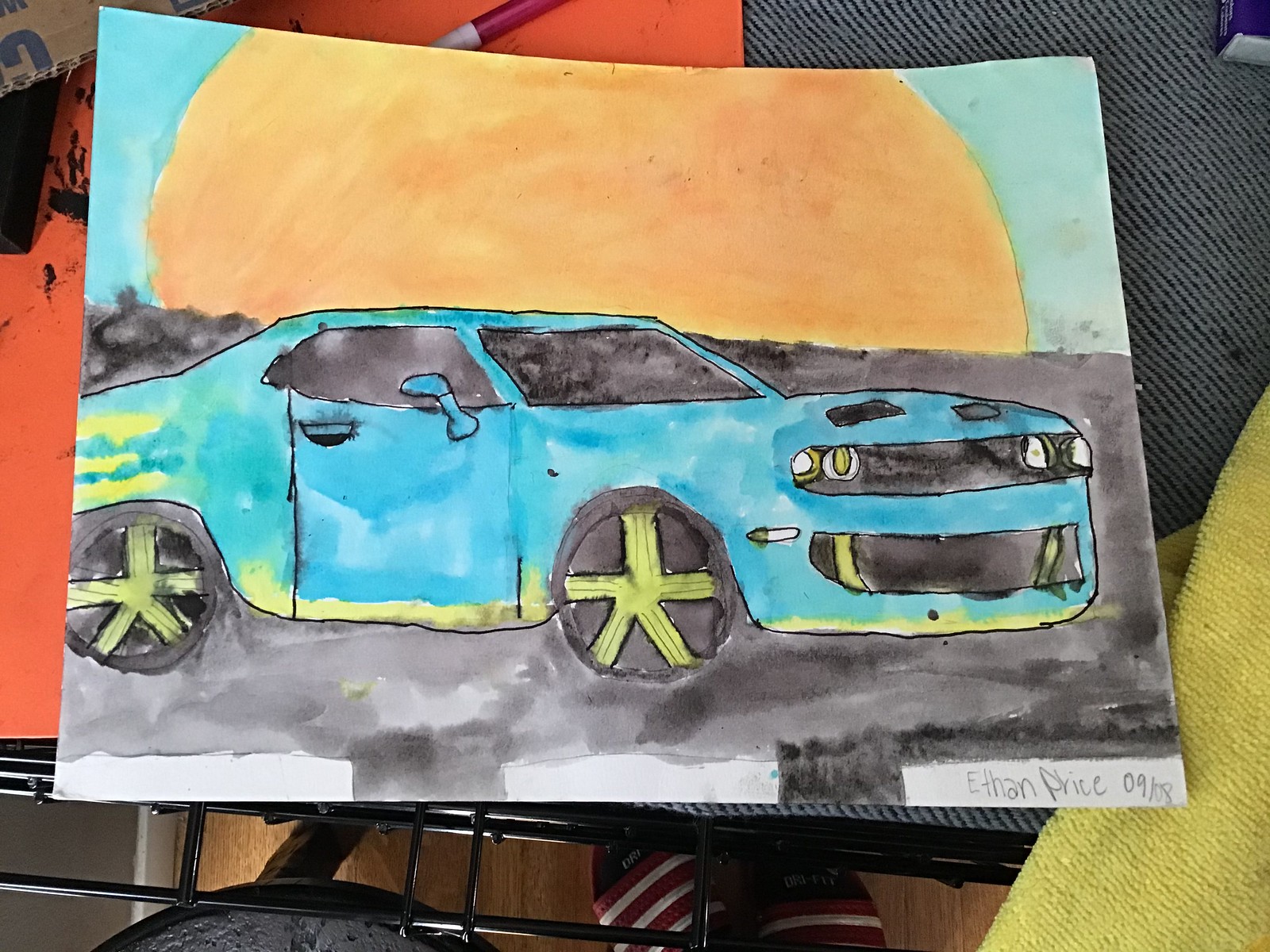This image captures a whimsical watercolor painting, likely created by a student in grade school or high school. The focal point is a light blue car, reminiscent of a Dodge Charger, positioned on a black roadway. The car is oriented from right to left, exposing its passenger side and showcasing black tires with distinctive yellow hubcaps. The vehicle features vibrant yellow accents on its door edges, trunk, and hood, along with four white headlights and a visible grille. Above this scene dominates a large, brilliant orange sun, either setting or rising, against a blue sky. Yellow stripes are subtly integrated into both the car and the road below. Below the main artwork, the signature "Ethan Price 09/08" is clearly visible, suggesting the date September 8th or the year 2008. The painting appears propped up in a classroom setting, with glimpses of gray and orange colors, possibly decorations or classroom materials, and a yellow item at the bottom left corner.